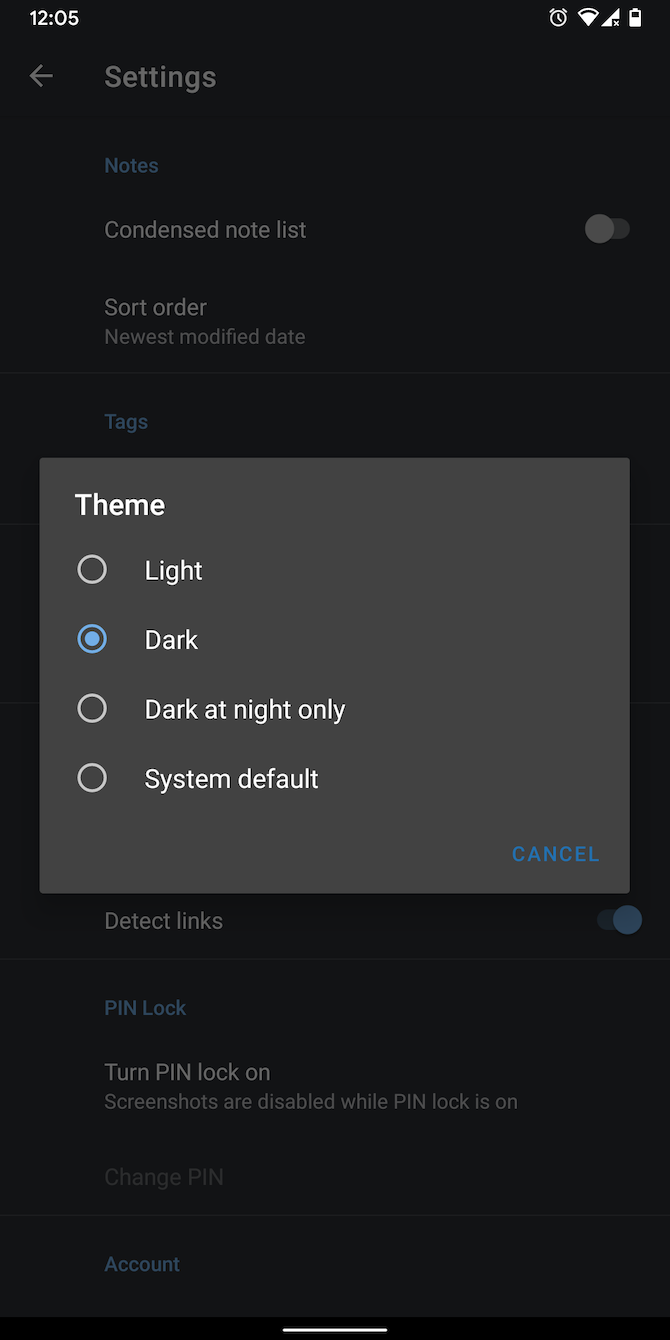The screenshot captures the settings area of a phone, focusing on a pop-up menu for theme selection. 

In the top right corner, the battery icon is vertically oriented and approximately 60% full, colored white inside. Left of the battery icon, a phone signal strength icon shows full bars with a small 'X' at the bottom right, indicating some connectivity issue. Next to it, a Wi-Fi signal strength icon is nearly full, with only one bar missing. An alarm clock icon is also visible in this cluster of status icons.

On the top left, the current time displayed is 12:05. 

The central part of the image features a pop-up menu. At the top left of the pop-up, the word "Theme" is displayed. Below it, four circles, resembling bubbles, are aligned vertically. 
- The first bubble is labeled "Light."
- The second bubble, labeled "Dark," is checked and filled with a blue color.
- The third bubble says "Dark at night only."
- The fourth bubble is labeled "System default."

At the bottom right of this pop-up, the word "Cancel" appears in blue.

In the background, the word "Settings" is prominently displayed at the top middle. Below it, a list of various settings options is partially visible, including options like "Condense," "No list," "Sort order," and "Turn pan lock on."